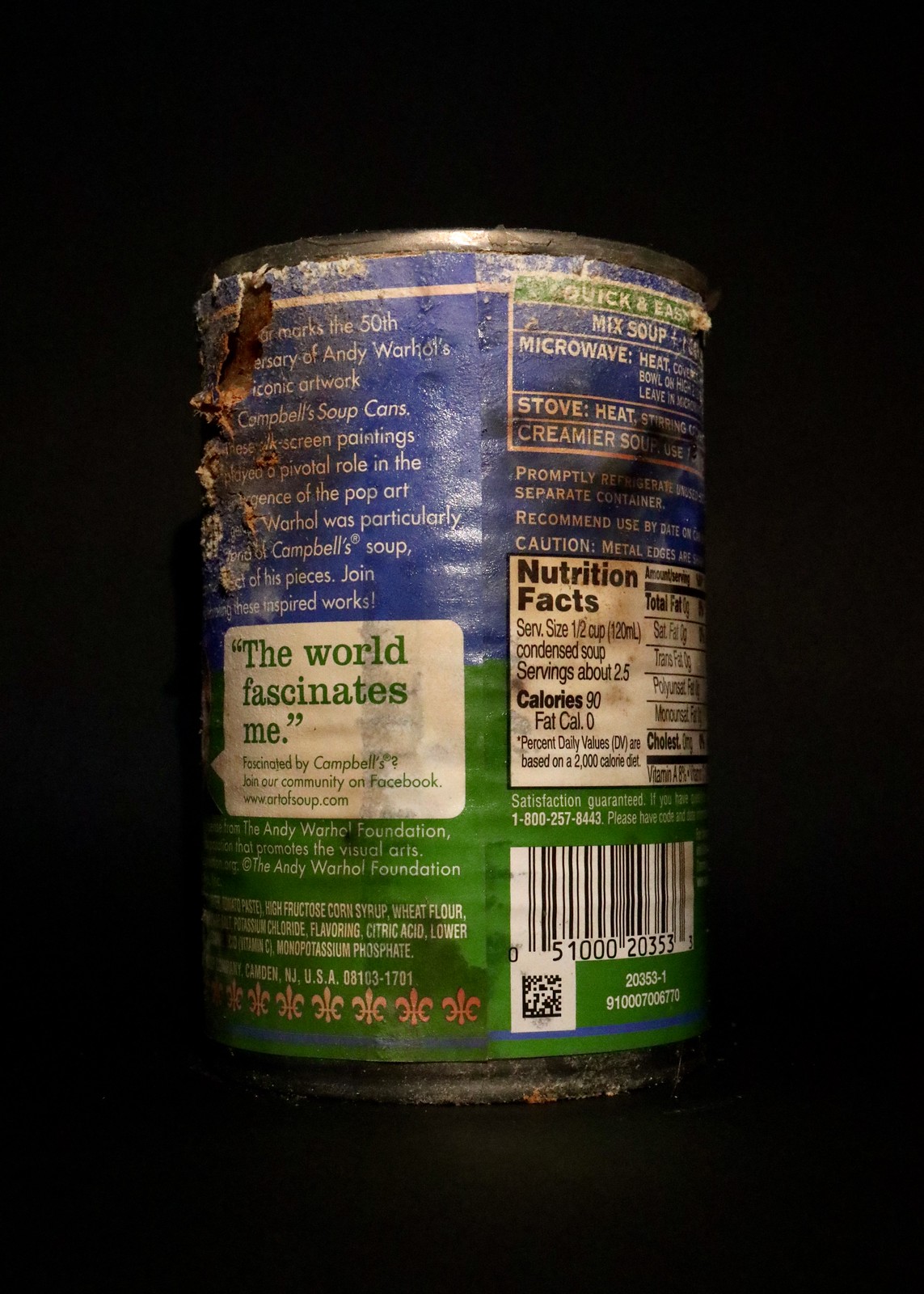This photograph showcases an old, distressed can of soup set against a completely black background with no shading or gradient. The can's label is heavily stained and deteriorated, displaying dirty and rusty spots across its surface. In the upper left corner, there is a noticeable tear in the can's label, exposing a brown, rusting area beneath where the blue of the label has worn away. Despite its distressed condition, the label still retains some color, featuring a blue section at the top with faded white print that is difficult to decipher. 

The bottom portion of the label is green with more white print. Notably, a white word bubble reads, "The world fascinates me. Fascinated by Campbell's. Join our community on Facebook, www.artofsoup.com." In the bottom right corner of the label, there is a UPC code and a QR code intact. The image highlights the aged and weathered state of the can, suggesting its historical or artistic significance.